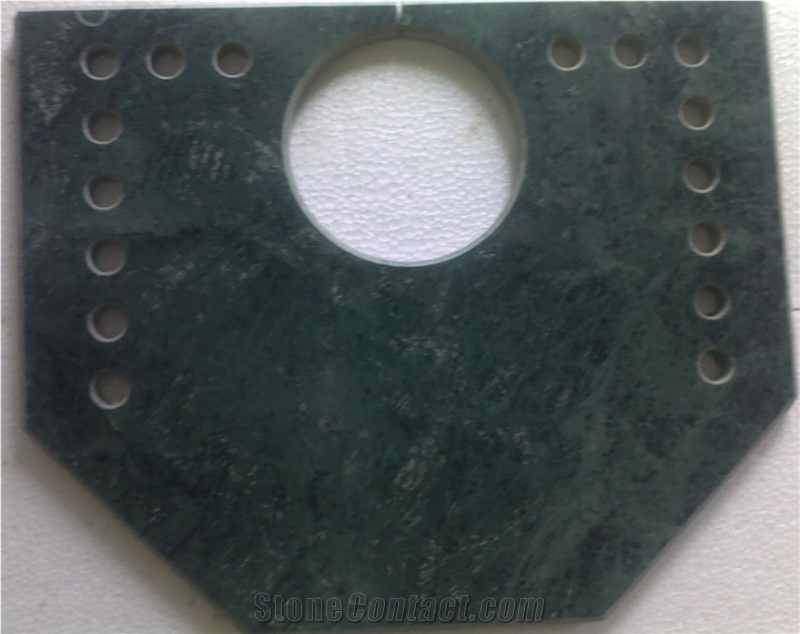This photograph captures a dark metal object, possibly used in engineering or machining, resting on an off-white table. The object is roughly pentagonal and flat, resembling a metal jig or plaque. Dominating the center is a large cut-out circle with ridged edges, surrounded symmetrically by smaller holes: three at each bottom corner and six running vertically up each side. The material appears to be a thick metal plate, estimated to be between three-eighths to half an inch thick. A faint watermark at the bottom reads "stonecontact.com," suggesting a possible connection to stone tools or materials. In the background, a light beige wall adds contrast to the dark metal object in the foreground.